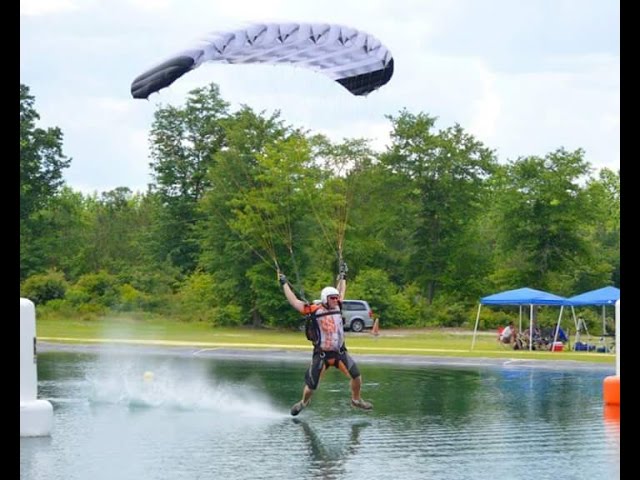In this vibrant color photograph, a man is captured mid-action while parachuting towards a pond, situated in what appears to be a public park. The man, outfitted with a black and white parachute, wears a helmet, sunglasses, gloves, and knee-length gray shorts. His arms are extended, gripping the parachute ropes as his right foot skims the water, creating a dynamic spray. To the right, in the mid-background, there are two blue-topped, 10-by-10 tents with four support poles each. Under one of these tents, several people, possibly a couple, are seated near a few coolers. The grassy area they are on extends to a backdrop of numerous trees, adding a natural enclosure to the scene. A gray van is parked in the distance, blending with the environment. On the lower left of the image, an unidentified white object floats on the water's surface. There’s also a camera on a tripod set up nearby, hinting that the event might be part of a formal or informal competition, as suggested by potential markers in the pond indicating landing zones. Framing the entire image are vertical black bars on both the right and left edges.